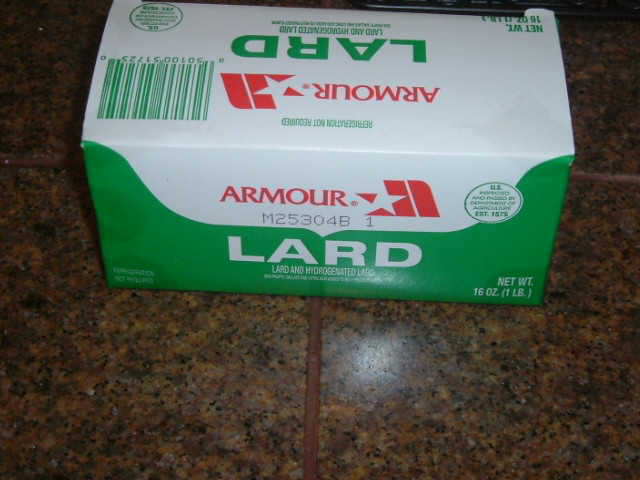The photograph depicts a rectangular cardboard container of Amour brand lard. The container is placed on a dark brown, mottled granite surface, which could be either a floor or a countertop. The prominent Amour logo, rendered in red, features a stylized letter 'A' with a white star cutout in its center. The bottom part of the box is green and prominently displays the word "LARD" in large white letters.

Beneath this, there is smaller white text indicating that the product is lard and hydrogenated lard. The net weight is also listed, detailing the contents in both ounces and pounds. On the top right corner of the box's lid, a large green barcode is visible, along with the instruction "Refrigeration Not Required," explaining that the hydrogenation process prevents the lard from melting or going bad without refrigeration.

The box has a flip-top lid, and although the photograph shows the backside, it suggests that opening the lid from the front would reveal the lard bricks inside, likely packaged similarly to butter. This product is presumably intended for cooking or frying, making it suitable for use in commercial kitchens or catering operations where such large quantities would be necessary.